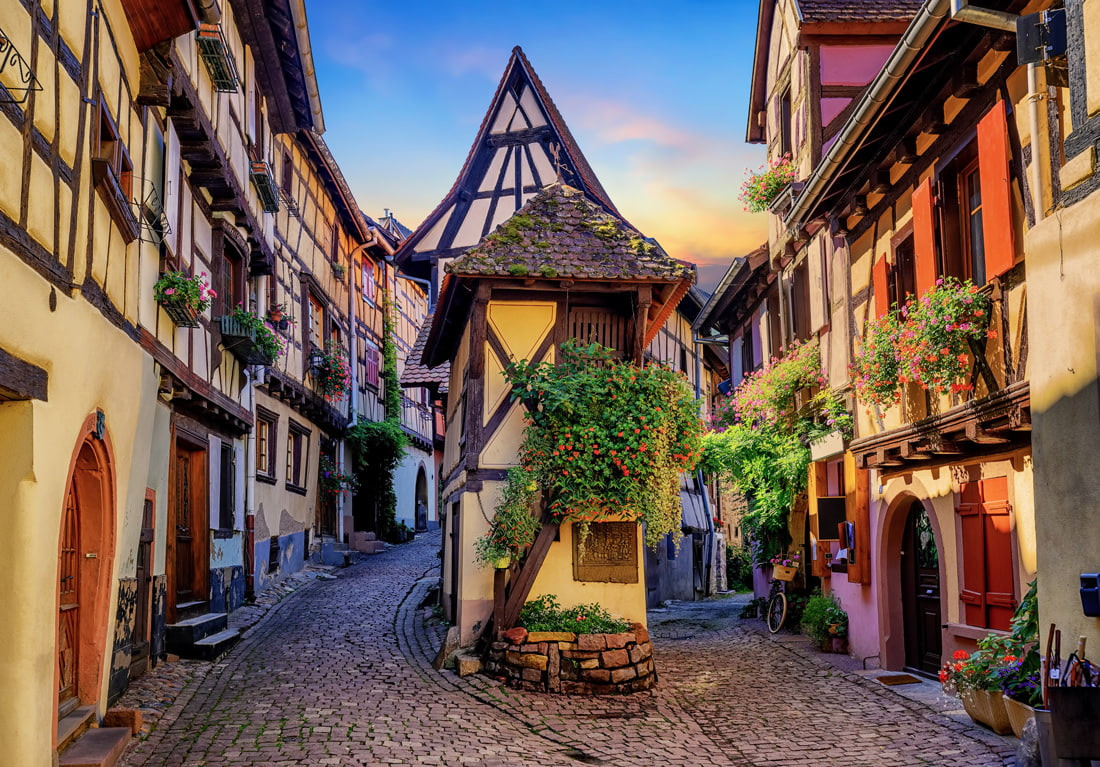This image showcases a picturesque cobblestone street in a charming, quaint European village, evoking the traditional half-timbered architecture of regions in France and parts of Germany. The buildings lining the street are adorned with colorful façades and exposed timber framing, with their windows overflowing with vibrant flower boxes in hues of pink, red, and green. At the heart of the scene, a distinctive building juts out into the street. This building features a triangular upper portion supported by a narrow base, and its exterior is covered in lush greenery and flowering plants that climb the walls and encircle the doorway. 

The buildings, three in total, are painted and each trimmed with brown, featuring orange doors and shutters. The street is flanked by flower beds and small brick gardens, with trees bearing red blooms adding to the flora. Upper windows display hanging flower baskets and houseplants, with additional plants on the ground level. The sky above is a serene blue with hints of yellow and pink near the triangular rooflines. The image captures an old-world neighborhood atmosphere, absent of inhabitants, yet alive with the vibrant details of nature and traditional architecture.